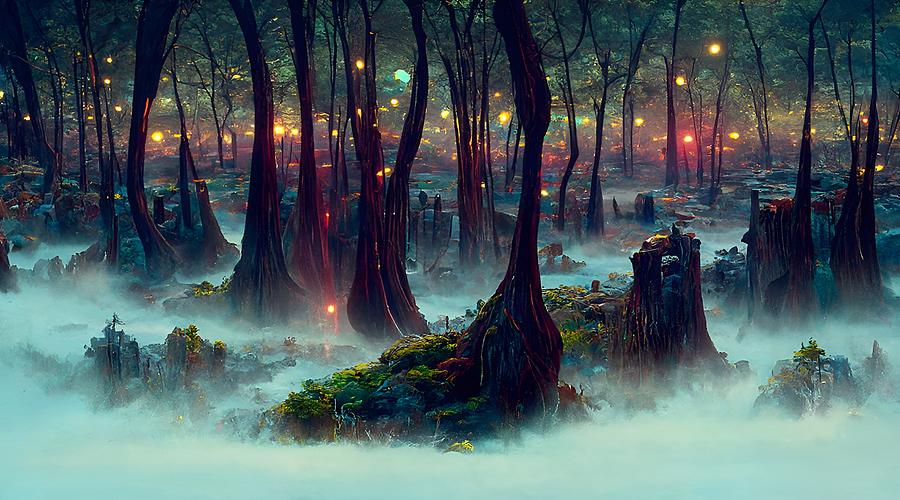The image appears to be a computer-generated or artist-rendered forest with a mystical, fantasy-like atmosphere. The scene is dominated by strange, reddish, and wispy trees that curve upwards, creating an almost otherworldly canopy. The ground is covered in a thick, white fog that adds an eerie and mysterious feel to the setting. The background is illuminated with numerous circular lights in shades of yellow, white, and red, resembling fireflies or distant lanterns that suggest the presence of a hidden village or camp. These lights contribute to the notion of people or creatures living within the base of these eerie trees, enhancing the scene's magical aesthetic. The overall ambiance suggests a nighttime setting, reminiscent of enchanted forests found in fantasy stories like Harry Potter or Lord of the Rings.